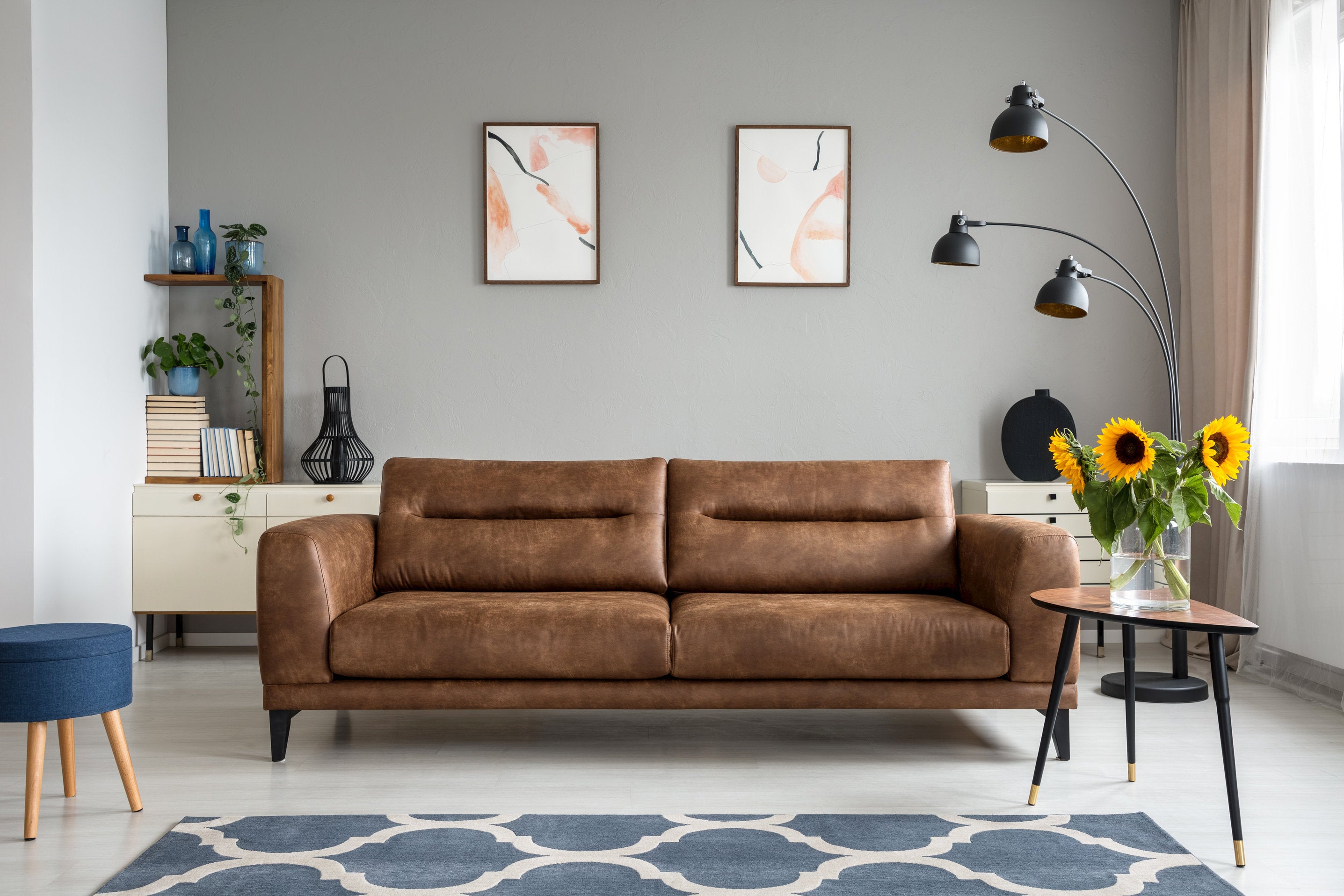This stock photo captures a stylish, modern living room with meticulous attention to detail. Central to the composition is a large, brown leather sofa, characterized by straight-line tufting on the back cushions. To the left of the sofa is a blue stool with tripod legs made of blonde wood, while to the right stands a distinctive three-armed reading lamp with black, powder-coated, steel shades that arc gracefully over the seating area. Adjacent to the lamp, a triangular table with black tripod legs and a wooden top supports a clear vase filled with water and bright yellow sunflowers, complete with stems and leaves. The background features a modern bookcase set atop a sleek, white laminate sideboard which has brown wood knobs. The bookcase is filled with books, blue vases, and additional plants, enhancing the room's contemporary vibe. The light grey walls are adorned with abstract modern art paintings featuring red splotches and black lines. The room is anchored by a beige and blue geometric rug on the light grey hardwood floor, which adds a cohesive touch to this aesthetically pleasing environment. A large window with ivory curtains filters natural light, completing the serene ambiance of this living space.